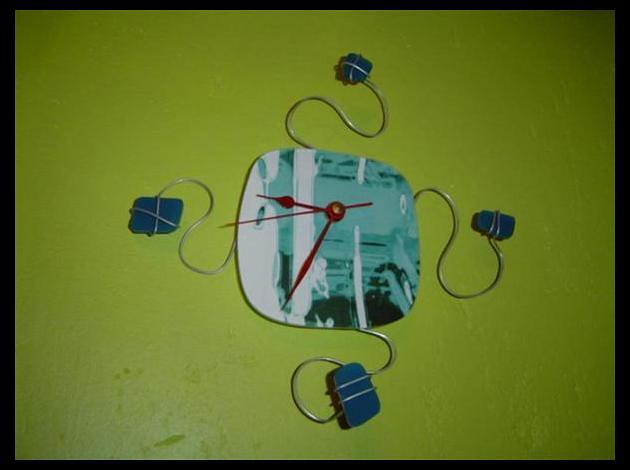The image features a square clock with rounded edges centered against a pea green background bordered by a black outline. The clock's face displays a light turquoise color with varying shades of dark turquoise near the bottom, center, and right side, forming a distinctive pattern with a rounded area of dark turquoise at the bottom. There is a white streak running down the center and a thicker white streak towards the left, with the left side predominantly colored in white.

The clock's hands are all red: the minute and hour hands are thick, while the second hand is thinner. From the top, bottom, and each side of the clock, a silver rope extends outward, symbolizing connectivity. Each rope wraps around a small blue element: the top rope ends in a smaller blue shape, the left and bottom ropes wrap around slightly larger blue squares, and the rope on the right ends in a smaller blue piece. The exact purpose and material of these blue elements remain unclear, adding an element of intrigue to the design.